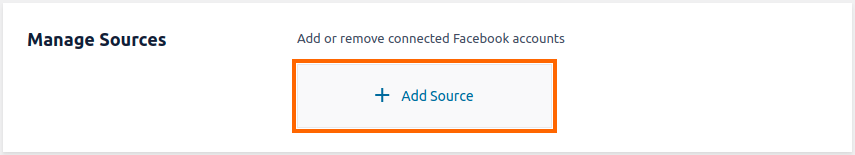This image captures a webpage titled "Manage Sources," prominently displayed in bold black text at the top. Below this header, the text "Add or Remove Connected Facebook Accounts" provides further instructions. Dominating the center of the image is a large rectangular box outlined in gray with an additional orange highlight around it. This box features a white background and contains the phrase “Add Source” centered within it, written in blue text accompanied by a blue plus sign. The overall design suggests interactivity, indicating that clicking the "Add Source" option would prompt a secondary box for input, allowing users to add or remove Facebook accounts. The structured layout and clickable elements imply that this interface is part of a settings page typically found on a computer.